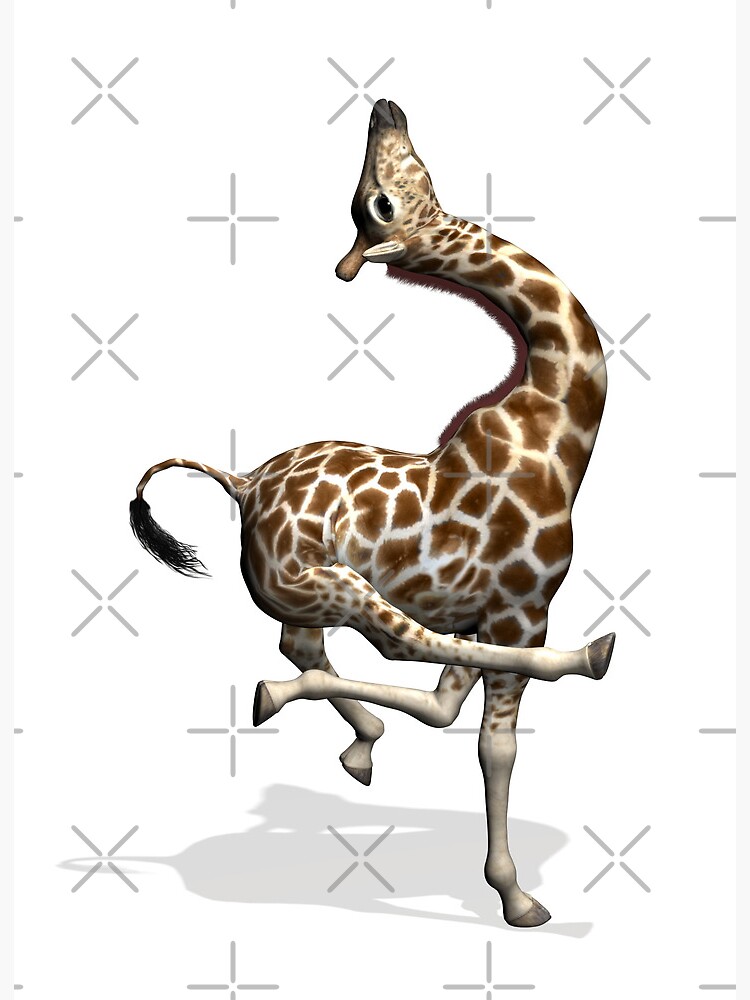The image features a computer-generated, cartoonish giraffe that appears to be dancing joyfully on a white background adorned with gray patterns of Xs and plus signs. The giraffe is primarily brown and beige with distinctive white feet and a brown nose. Its body is oriented to the right side of the image, while its neck is dramatically curved into a backward C, causing its head to face upwards, almost as if it is looking at the ceiling. Its legs are in various dynamic positions: one front leg is straight and grounded, another is kicking backwards, and one of its back legs is crossed over the front leg. The giraffe’s vibrant pose is further animated by its uplifted tail, casting a playful shadow on the backdrop. This whimsical and entertaining portrayal, devoid of text, resembles an engaging card or poster, capturing the essence of a dancing giraffe in a lively, exaggerated form.